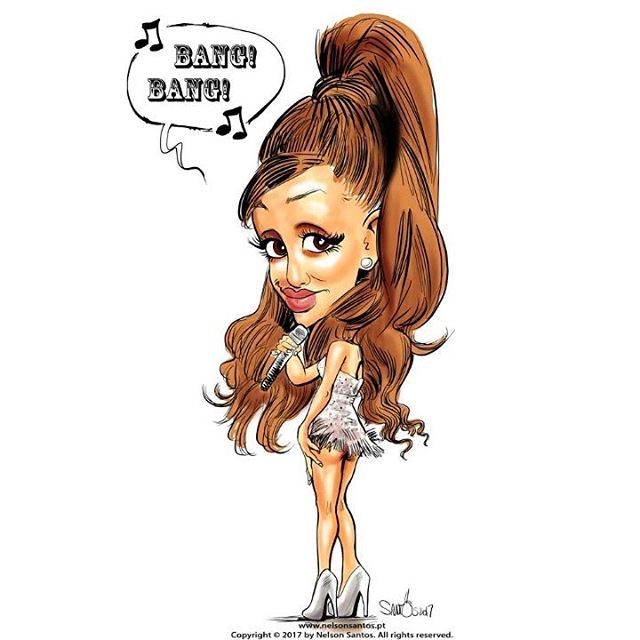The image is a colorful, portrait-oriented caricature illustration by Nelson Santos, copyright 2017. It depicts a young woman, likely the singer Ariana Grande, standing with her back mostly to the viewer while looking over her left shoulder and smiling. She has exaggeratedly large eyes and lips, and her long reddish-brown hair is styled in a high ponytail, cascading down to her bottom in ringlets. She is dressed in a short, skimpy, white fringed dress that reveals her bottom and wears tall white high heels. In her right hand, she holds a small microphone. Above her head, in the left corner of the image, there is a speech bubble with the words "bang bang!" in black Western font, accompanied by musical notes, suggesting she is singing. The artist's signature and website, www.nelsonsantos.pt, are present at the bottom of the illustration.